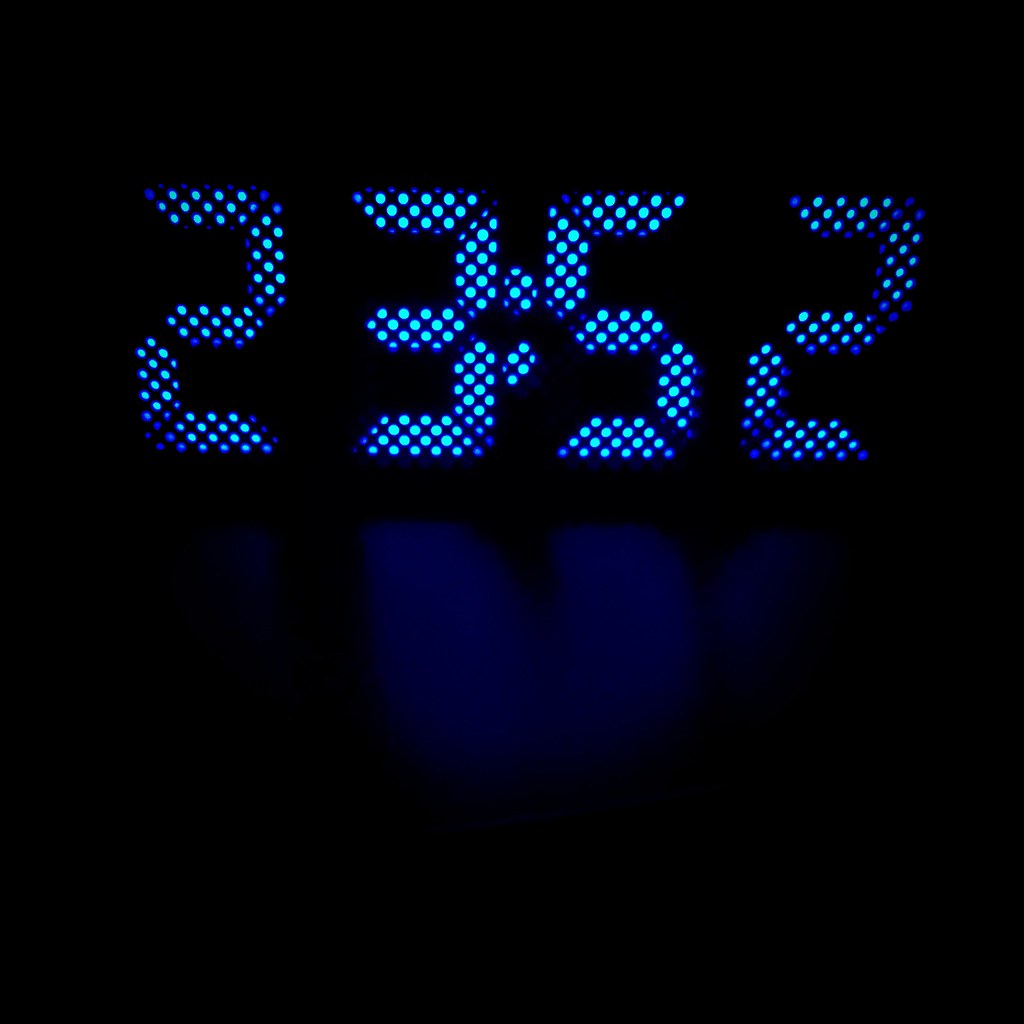This vibrant color photograph captures a nighttime scene with a digital alarm clock as its focal point. The background is entirely black, placing full emphasis on the illuminated display of the clock. The time is shown in large, clear, dark and light blue digital numbers, reading "23:52" in a 24-hour military format. A subtle blue glare from the display is visible on the surface below the clock, adding a touch of depth and dimension to the otherwise minimalist composition.